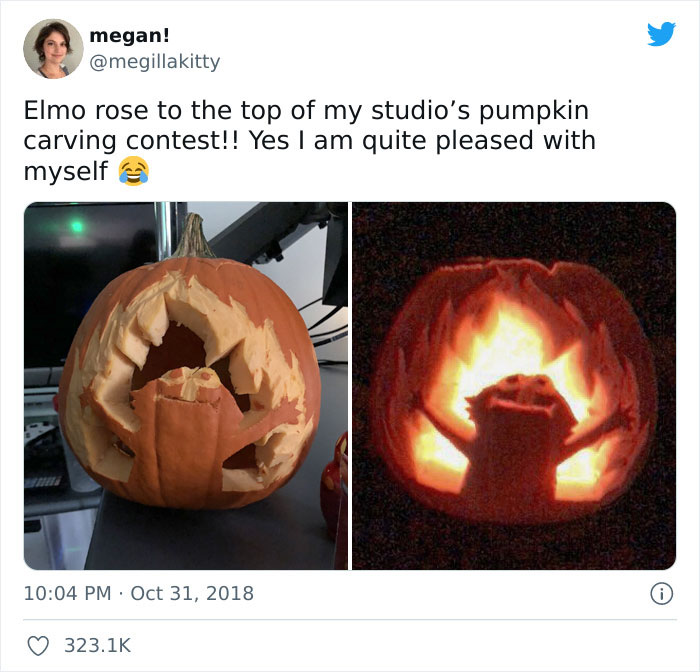**Twitter Post by Megan (@MegLaKitty)**

*Profile Picture: Megan with short brown hair, smiling and wearing a black and white top.*

---
Elmo rose to the top of my studio's pumpkin carving contest! Yes, I am quite pleased with myself 😆 

* (Left Image) - A intricately carved pumpkin features Elmo surrounded by flames, resting on a table. In the background, there are some computer wires, a green light, and a remote control. 

* (Right Image) - The same pumpkin illuminated in the dark, highlighting Elmo with his hands spread out and flames vividly glowing around him.

*Post Timestamp:* 10:04 p.m., Halloween, October 31, 2018

*Engagement:* 323.1K likes

---

*Twitter Bird Logo:* Aqua-colored in the right-hand corner.